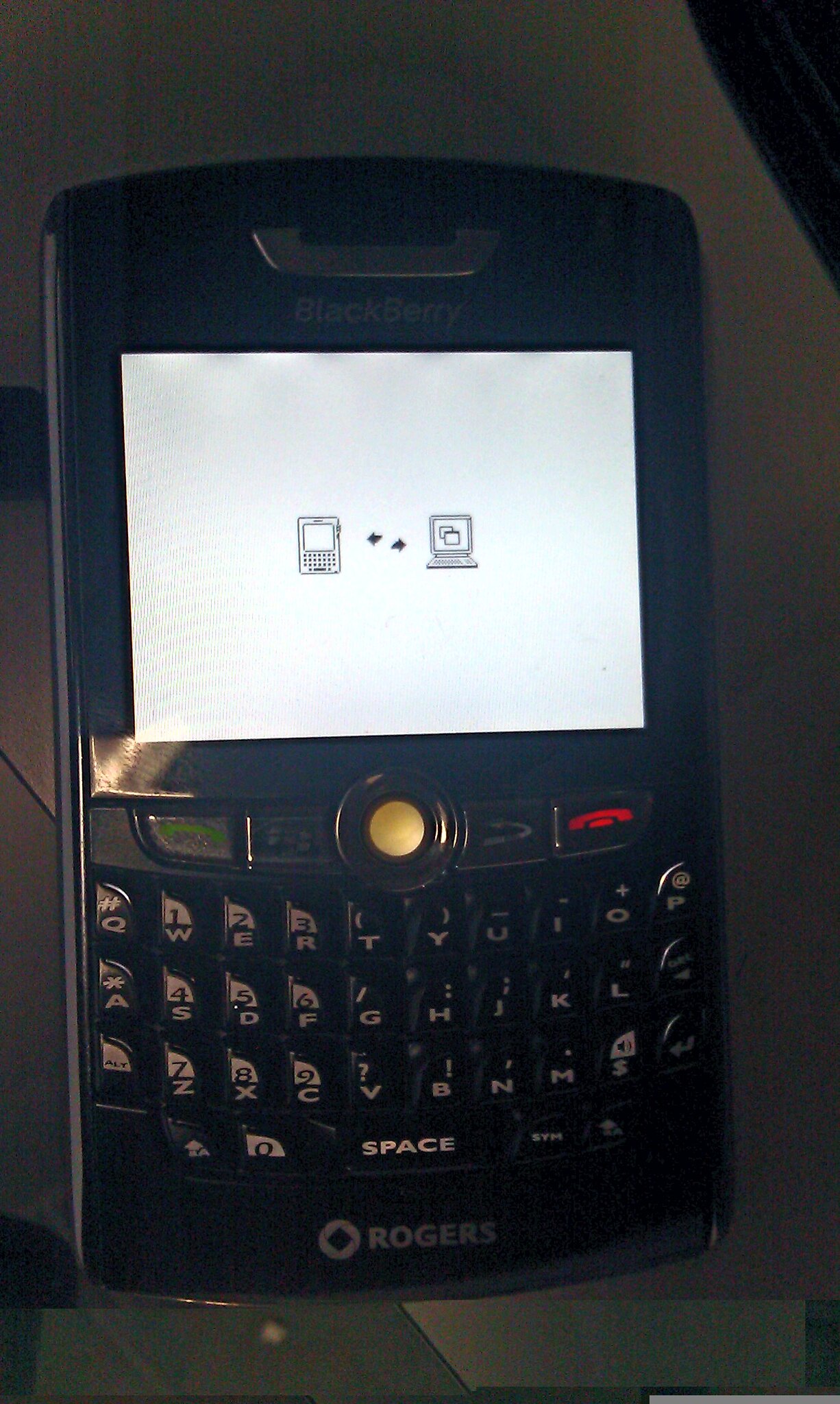The image displays a close-up of an older BlackBerry smartphone, characterized by its black exterior. Prominently featured at the top is a white screen displaying two icons—a laptop and a smartphone—suggesting data transfer between the devices, highlighted by arrows. Below the screen, the BlackBerry logo, resembling an upside-down phone receiver, is visible. Directly beneath the screen, there is a set of navigation buttons including a central gold button, flanked by a green call button and a red hang-up button. The lower portion of the device showcases a full QWERTY keyboard with alphanumeric keys and a space button at the bottom. The brand name "ROGERS" is inscribed at the very base of the phone. The backdrop of the image is a dark grayish hue.